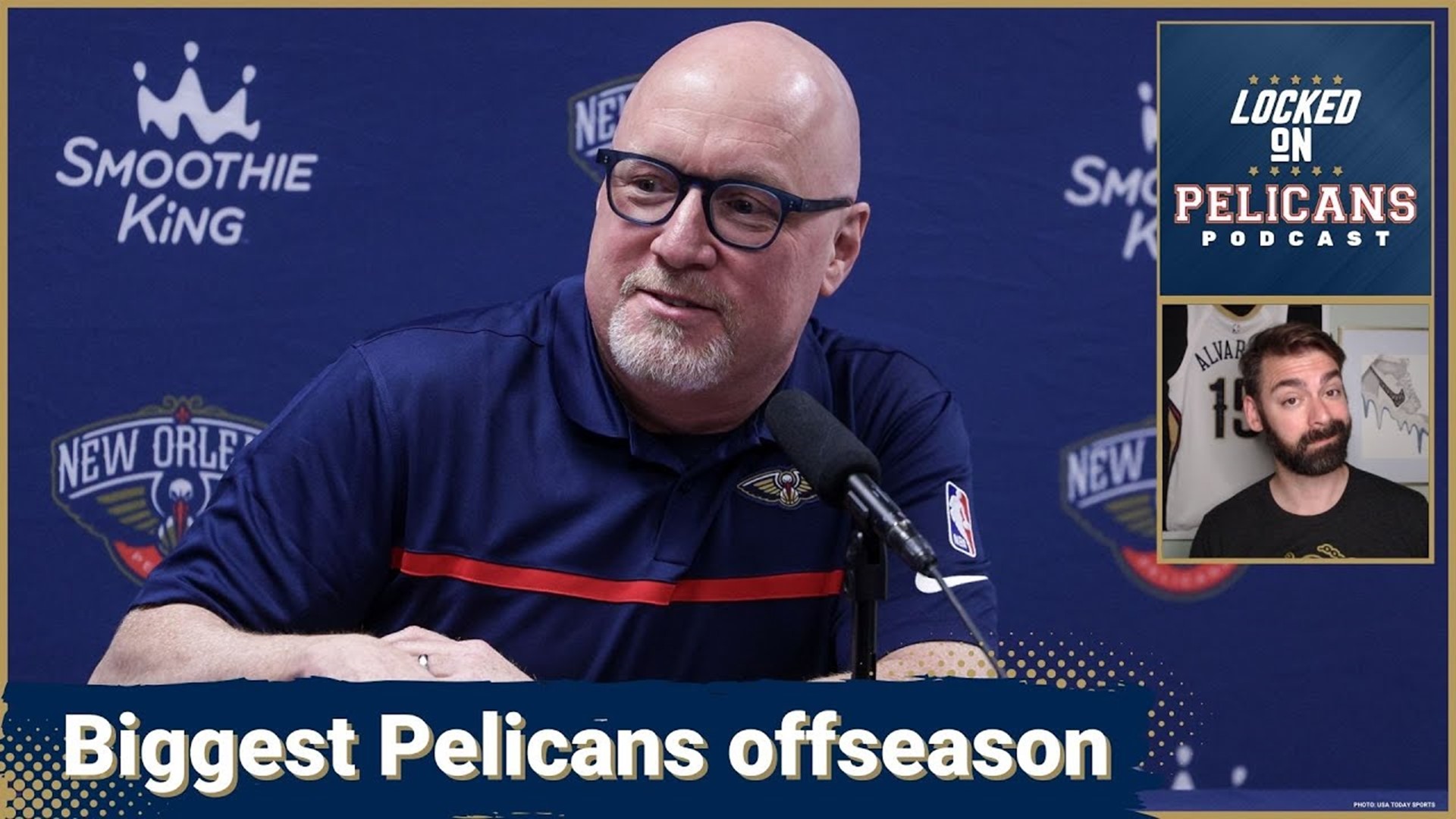The image is a rectangular screenshot, approximately six inches wide and three inches tall, featuring what appears to be an interview or podcast frame. It is bordered by a thin, light tan line. The setting has a plain blue background adorned with a light gray "Smoothie King" advertisement that features a crown above the text, and "New Orleans" written beneath, repeated across the backdrop from left to right and top to bottom.

In the center of the image, there is an older Caucasian man, likely in his 60s, sitting from mid-chest up. He is bald with black or blue glasses and has a graying mustache and beard on his chin. He is dressed in a blue collared polo shirt with a red stripe running horizontally across it, displaying both the Nike symbol and the NBA logo on the sleeve. Below him, a banner is displayed with white text that reads, "Biggest Pelicans Off-Season."

In the upper right-hand corner of the image, there is an inset rectangle outlined in gold and split centrally by a gold bar. The top half of this inset has white text that says, "Locked On Pelicans Podcast," and the bottom half contains a photograph of a younger man of Caucasian descent with brown hair, beard, and mustache.

This meticulously detailed composition suggests the man in the image is possibly involved in discussing the Pelicans' off-season activities on the "Locked On Pelicans Podcast."